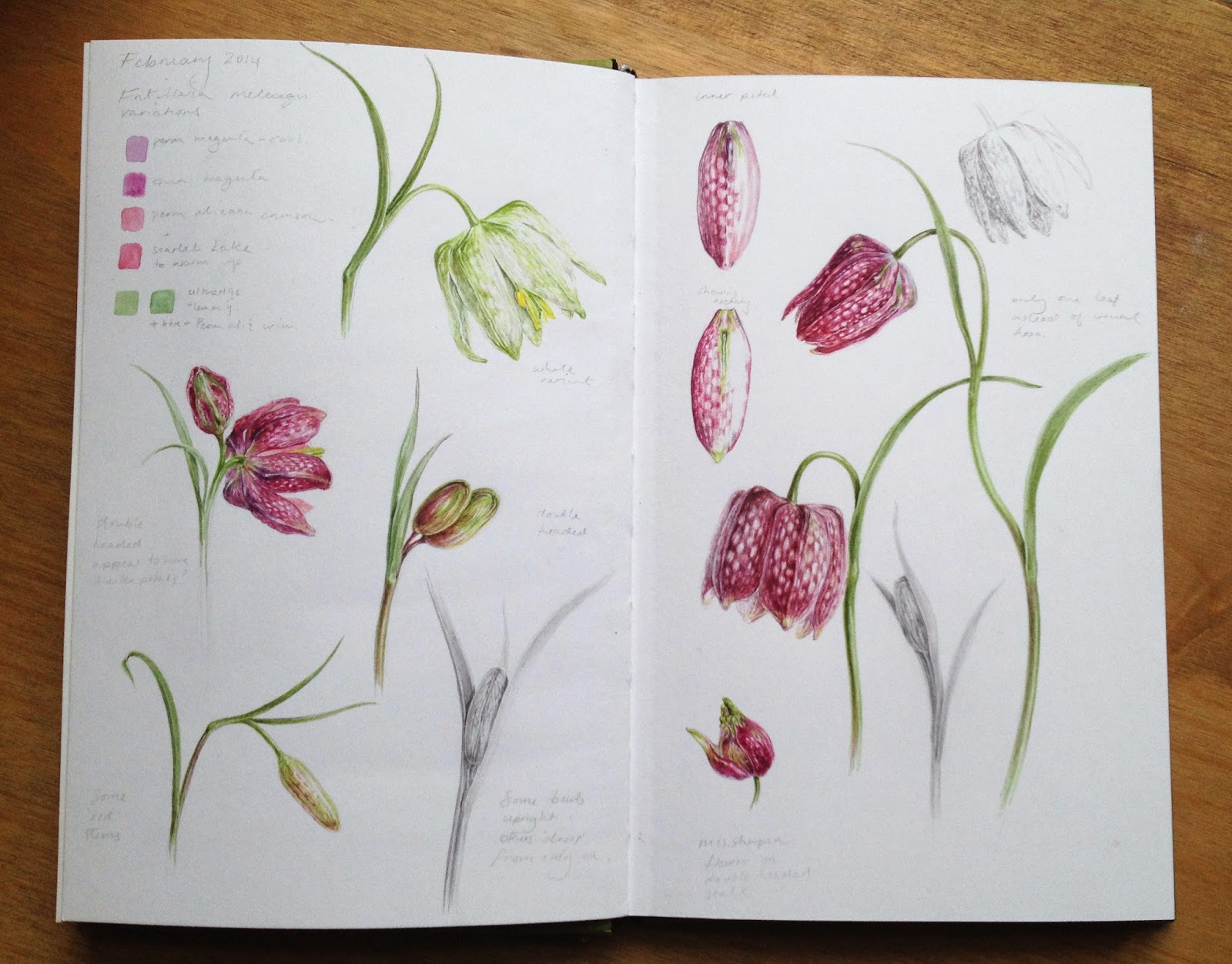This image features a top-down view of an open sketchbook with white pages that contain an array of detailed flower sketches. The left page prominently displays a color-coded legend at the top left, featuring squares in purple, darker purple, pink, red, light green, and dark green, each corresponding to specific shades used in the drawings, though the accompanying text is not readable. Below the legend, there are five distinct floral illustrations. The top left corner features a white flower, followed by a pink flower and two flower buds beneath it. On the bottom left is a yellow flower, with a black-and-white sketch of a flower bulb emerging from a stem at the bottom right. 

The right page primarily showcases sketches of various stages of a pink tulip's bloom. At the top right, there's a small black-and-white sketch of the tulip. Two flower buds in purple are drawn at the top left, while two blooming flowers are shown on the right side. The center of the right page depicts the flower facing downwards. Additionally, there are meticulously illustrated parts of the tulip, including the pink petals and flower buds at various stages of development. Some sketches focus on the tulip's structure and how it forms from buds to a fully opened flower.